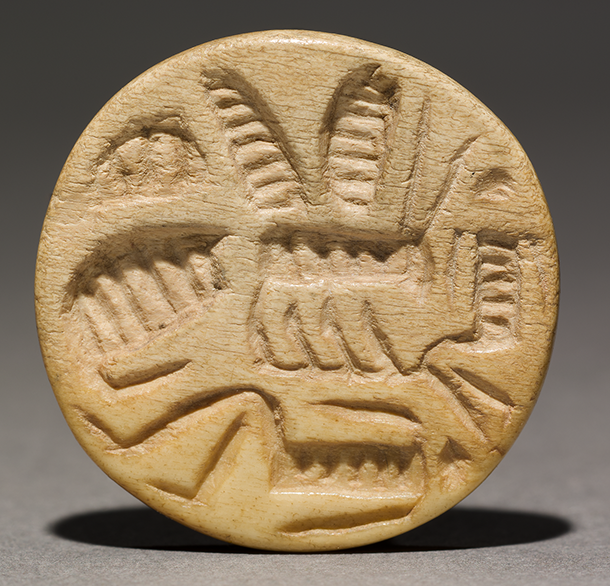The image depicts an ancient, round, creamy tan disc, likely made of clay or stone, standing on end against a gradient gray background. The object casts a black cylindrical shadow on the gray floor. The disc is meticulously engraved with numerous bean-shaped indentations, each carved with deep lines, suggesting a high level of craftsmanship. The bottom portion of the disc features a slight geometric pattern, indicating possible symbolic or decorative significance. The artifact appears well-preserved, standing out against the background with its smooth and detailed engravings, which may represent traditional or indigenous symbols. The variations in surface finish—smoother at the bottom—could imply a design choice or wear over time, emphasizing its antiquity and cultural value.